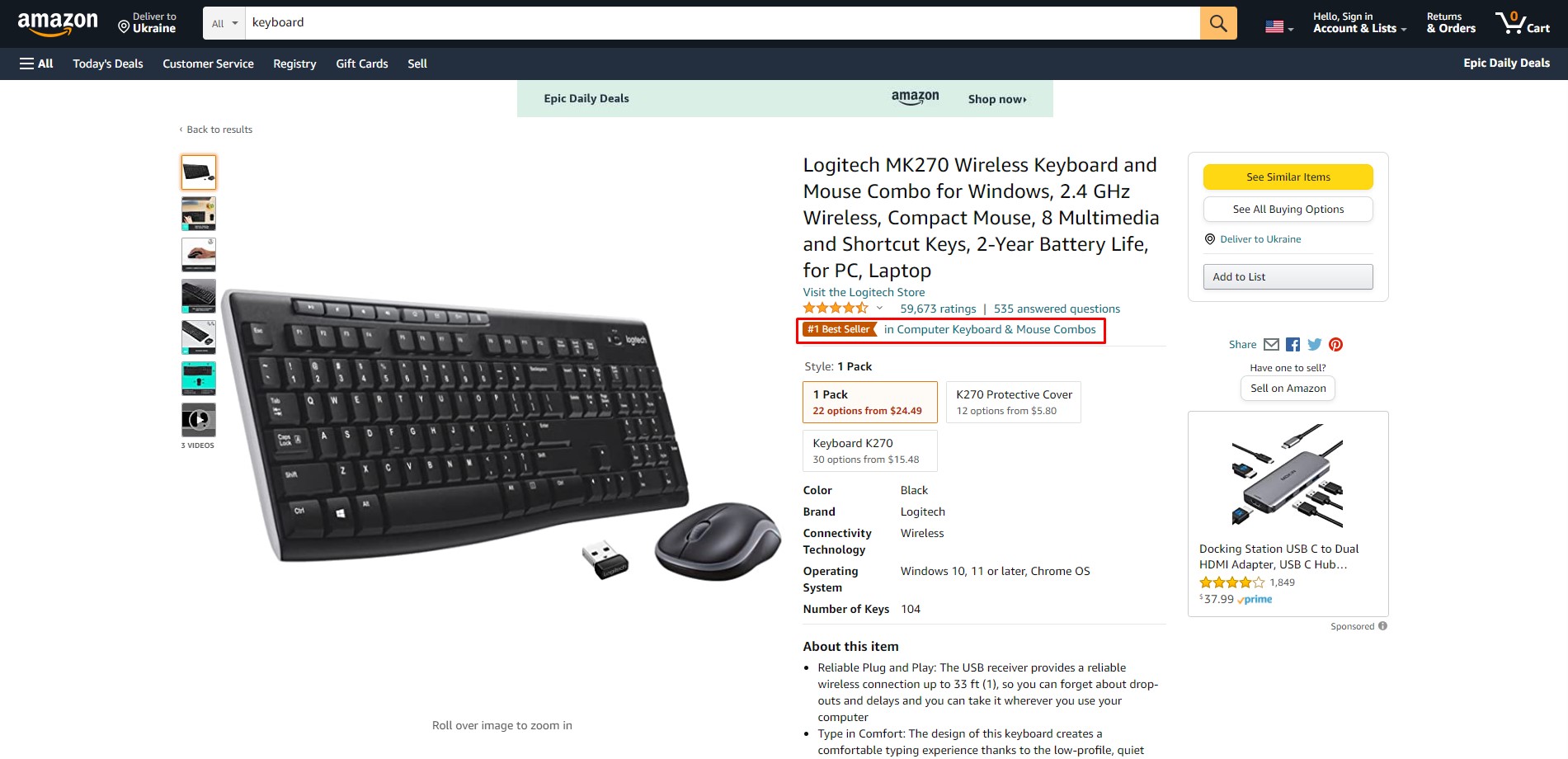The image showcases the Amazon desktop shopping website, featuring a detailed listing for a keyboard. Starting from the very top, the webpage includes a menu bar adorned with the Amazon logo on the left side, followed by a location icon, and a large search bar where the word "keyboard" is entered. On the right side of the bar, there are options to select the country, a sign-up button, a 'Returns & Orders' button, and a cart icon.

Beneath this primary navigation, a secondary menu offers links to "All," "Today's Deals," "Customer Service," "Registry," "Gift Cards," "Sell," and "Epic Daily Deals." Below these options, the main content area centers on the search result for the keyword "keyboard."

The central image displays a black Logitech MK270 wireless keyboard and mouse combo, prominently positioned against a white background. The set includes a keyboard, a mouse, and a small USB receiver. To the left of the main image, there are thumbnail images that can be clicked to enlarge and provide different views of the product.

To the right of the keyboard image, there is a detailed description of the listed item: "Logitech MK270 Wireless Keyboard and Mouse Combo for Windows — 2.4 GHz Wireless, Compact Mouse, 8 Multimedia and Shortcut Keys, Two-Year Battery Life for PC and Laptop." Below this description, the star rating of the product and the number of reviews are displayed, along with additional product details.

At the top right corner of the description section, there are purchasing options available. Below this, there are suggested add-on items compatible with the keyboard combo, such as a USB station or HDMI adapter.